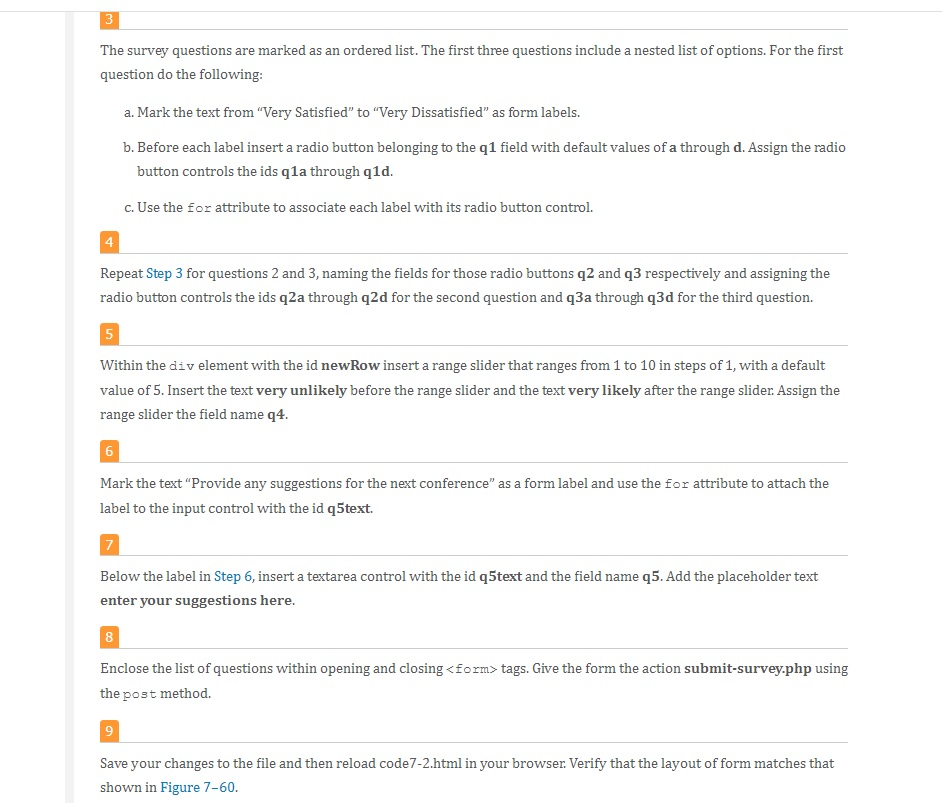**Detailed Caption:**

The image is a screenshot of a structured web page with a white background, divided into several sections by lines for clear separation. On the top left, there is an orange box with a white number "3" inside. Directly beneath this, a set of instructions is outlined in dark gray text.

The first instruction specifies that survey questions are presented as an ordered list. The initial three questions contain nested lists of options. For the first question, detailed steps include marking the text ranging from "very satisfied" to "very dissatisfied" as form labels. Each label is preceded by a radio button associated with the "Q1" field, defaulting to values from A to D. Notably, the characters "A" and "D" are highlighted in darker gray, indicating emphasis. To the right of these instructions, there are additional directives to assign IDs from "Q1A" to "Q1D" to these radio buttons, these IDs are also shown in darker gray for emphasis. The instruction concludes with associating each label with its respective radio button using the "for" attribute, presented in lighter gray.

Further down the page, another orange box houses a white number "4." Below this, an instruction in dark gray states to repeat the steps of step three. The steps are reiterated for questions two and three, assigning IDs as "Q2A" through "Q2D" and "Q3A" through "Q3D" respectively, all described in a lighter gray color.

Continuing downwards, an orange box with a white number "5" directs in dark gray to configure a DIV element with a new ID, "new row," in darker gray. Instructions include inserting a range slider ranging from 1 to 10 with steps of one, defaulting to a value of five, and placing the text "very unlikely" before the slider and "very likely" after it. The slider is to be named "Q4," which is highlighted in darker gray.

Beneath, another section begins with an orange box holding a white number "6." This part instructs users to mark text reading "Provide any suggestions for the next conference" as a form label and attach this label to an input control identified by "Q5 text," with all text in gray and the ID in darker gray.

Lastly, an orange box features a white number "7." Below this, instructions, initially in dark gray and then in blue, describe inserting a text area control with the ID "Q5 text" and field name "Q5." The placeholder text "Enter your suggestions here" in darker gray is to be included within the text area.